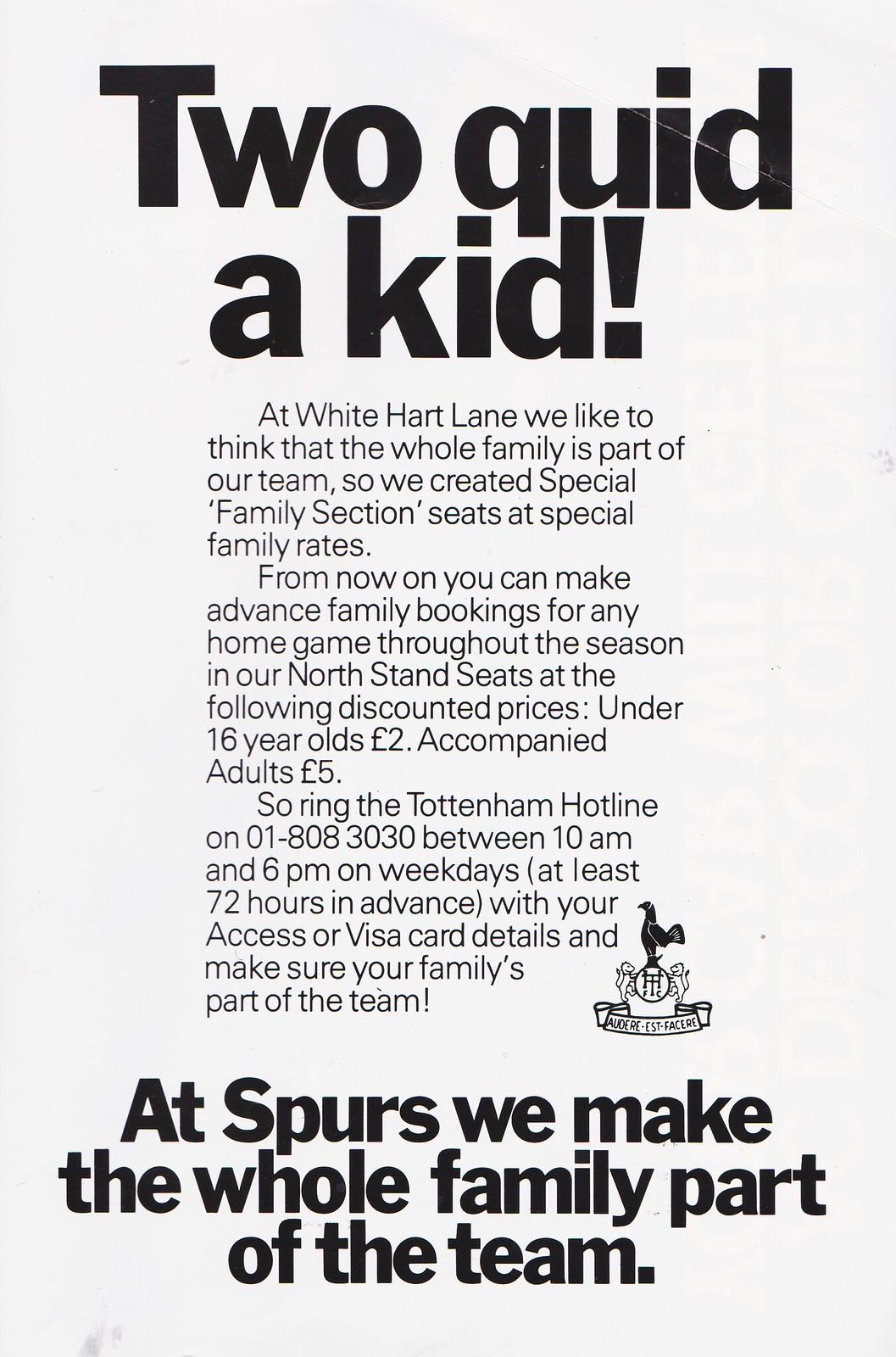The image is a vintage black-and-white advertisement from a magazine, promoting family-friendly seating at White Hart Lane. The top of the ad prominently features bold black letters that read "Quit a Kid," followed by smaller text stating, "At White Hart Lane, we like to think that the whole family is part of our team. So we created special family section seats at special family rates." It then explains that families can now make advance bookings for any home game throughout the season with discounted prices: £2 for children under 16 and £5 for accompanying adults. To book, one must call the Tottenham hotline at 01-808-3030 between 10 a.m. and 6 p.m. on weekdays, at least 72 hours in advance, and provide Access or Visa card details. The ad underscores the message with an emphatic statement at the bottom, in large black text: "At Spurs, we make the whole family part of the team." The ad also includes a logo on the right side, featuring a shield with "FC" and a cockerel perched on top, symbolizing the Tottenham Hotspur Football Club.